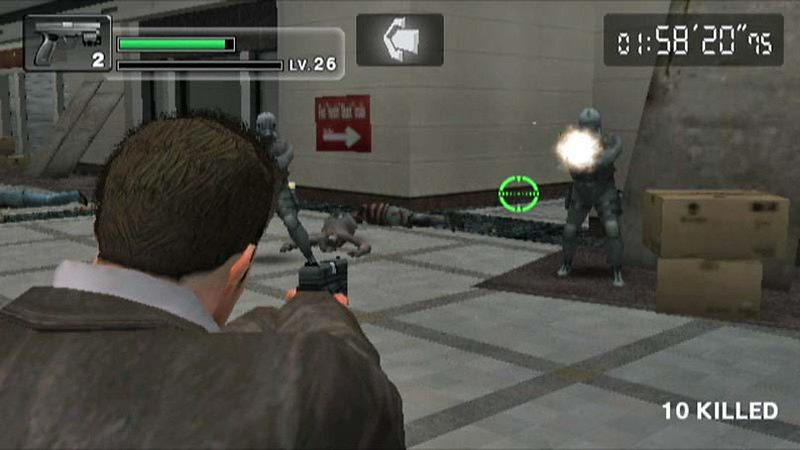In this screenshot from a first-person shooter video game, the perspective shifts to a third-person view, showcasing a tense combat scenario. The player character, a white male with brown hair, is clad in a brown jacket and is seen aiming a pistol with his right hand. He stands in a large, stark room with stone-like white walls and a grid-patterned gray tile floor. In front of him, two men are engaged in a fierce firefight. The enemy on the right side is actively firing his weapon, evidenced by a bright muzzle flash, and is positioned near some scattered cardboard boxes. The second adversary, on the left, also appears to be attacking. The aftermath of the battle is evident with several bodies strewn on the floor. A directional sign with an arrow pointing to the right is visible on the wall. The game's interface indicates at the bottom right corner that 10 kills have been achieved, while the top left corner displays the current weapon and progression points for leveling up.